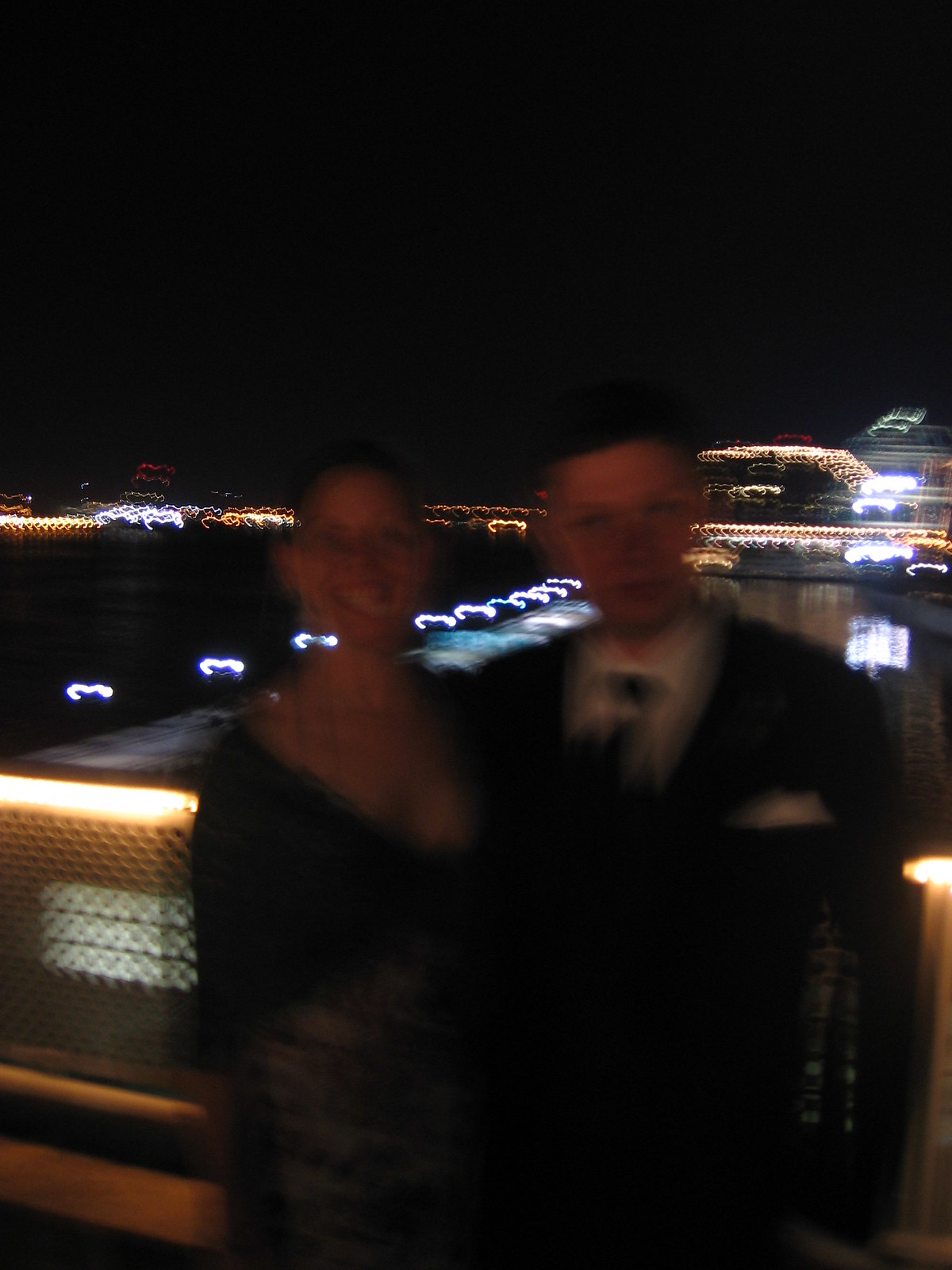In this blurry, nighttime color photograph taken outdoors, two individuals stand prominently in the foreground, their features slightly obscured by the lack of focus. On the right, a man dressed in a dark suit paired with a light-colored shirt and a dark tie gazes solemnly at the camera. A neatly folded handkerchief peeks out from his breast pocket. To his left, a woman, possibly wearing glasses, smiles warmly. She is dressed in a dark outfit, and her hair appears to be pulled back, giving her a polished look. Behind them, an array of blurred lights in shades of yellow and white create a bokeh effect, adding a hint of ambiance but providing no clear indication of the location due to the poor lighting and focus.